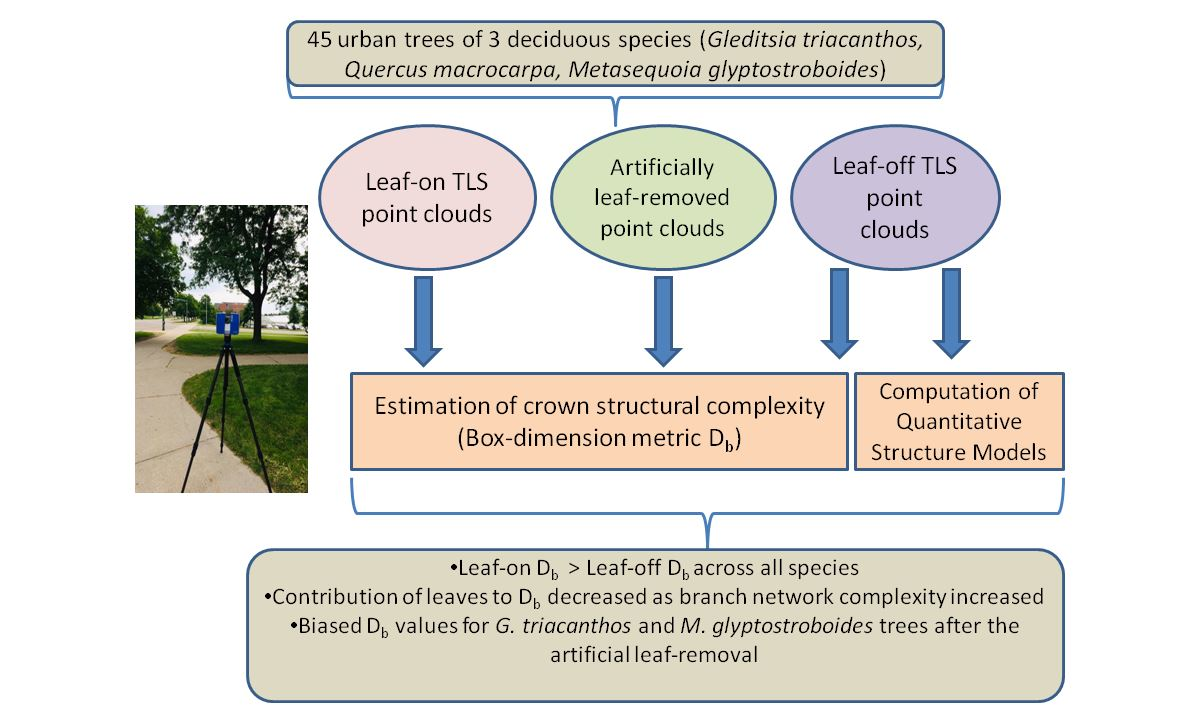The image depicts a detailed flowchart, likely from a textbook, illustrating an experiment involving 45 urban trees of three deciduous species: Gleditsia triacanthos, Quercus macrocarpa, and Metasequoia glyptostroboides (Latin names included in parenthesis). At the top, a title notes the species count and types, leading to three circles below. The left circle, in red, reads "Leaf on TLS point clouds," the middle circle, in green, states "Artificially leaf removed point clouds," and the right circle, in purple, indicates "Leaf off TLS point clouds." Blue arrows descend from each circle to orange boxes, which in turn point to a larger brownish box at the bottom. The orange boxes are labeled "Estimation of crown structural complexity," with the right one also mentioning "Computation of quantitative structure models." The brown box at the bottom summarizes results regarding the impact of leaf presence and absence on various structural metrics across species, noting changes such as "Leaf on D_b greater than Leaf off D_b" and contributions of leaves to the D_b metric. To the left of the flowchart, a small photograph shows an outdoor area with trees, a walkway, and a blue camera mounted on a black tripod, possibly used for surveying or photography in the experiment.